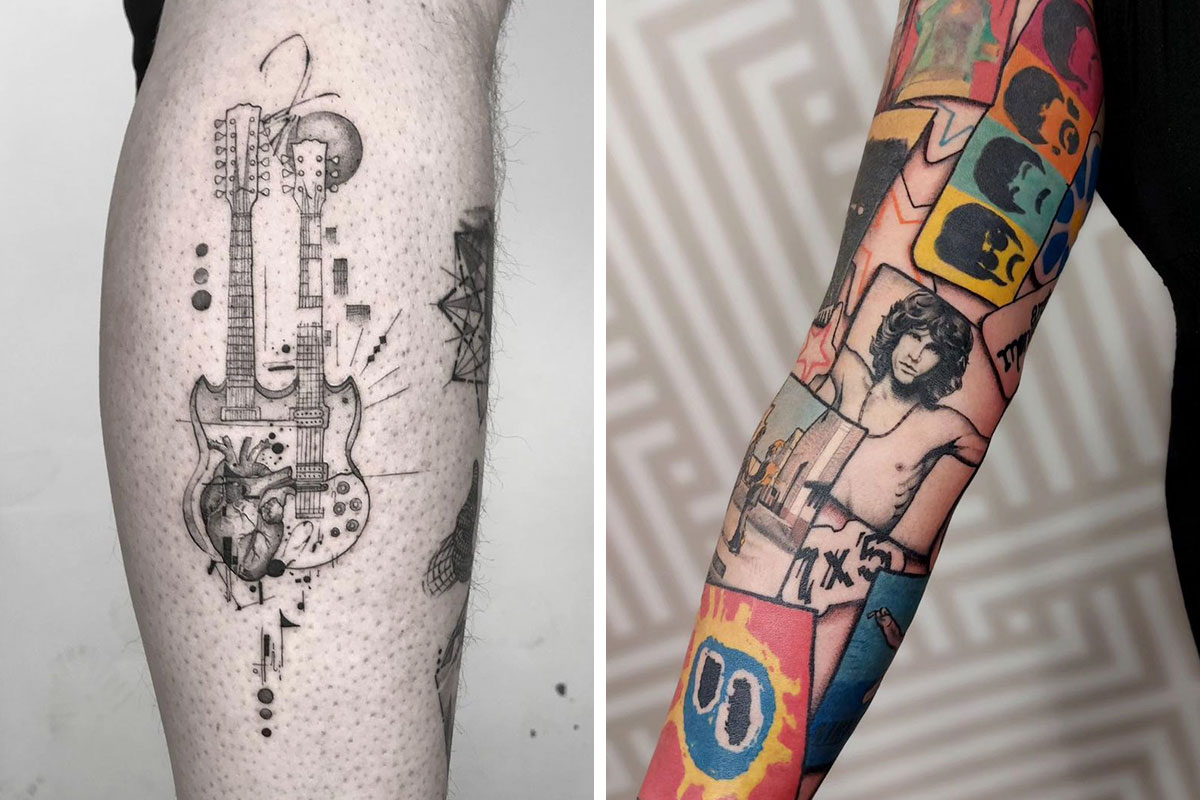The juxtaposed images depict intricately tattooed limbs, emphasizing a vivid celebration of music. The left photo features a pale human leg, specifically the section from the back of the knee to the ankle, adorned with a detailed black ink tattoo of two guitars intertwined at their strings, surrounded by musical notes and symbols. An intricately depicted heart appears at the base of one guitar, adding to the elaborate design. A subtle wall background highlights the tattoo's finer details. The right photo showcases an arm covered in a full sleeve of vibrant, colored tattoos. The artwork includes dynamic images of iconic rock music elements, prominently featuring a detailed portrait of Jim Morrison from The Doors, along with multiple faces and abstract patterns reminiscent of pop art. Various album cover concepts and numbers are also interwoven into the colorful collage, contrasting sharply with the monochromatic elegance of the guitar tattoo.